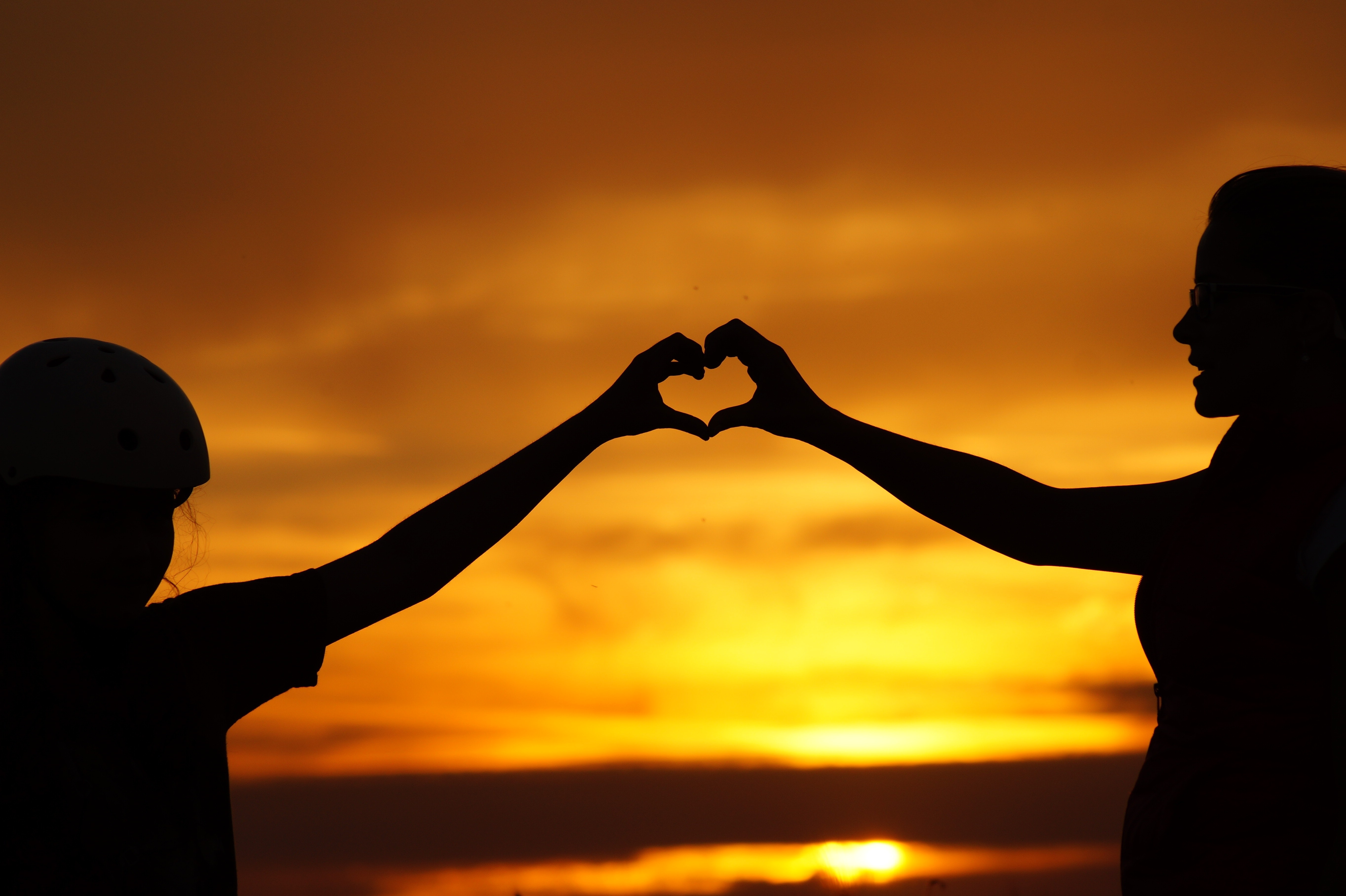In this captivating photograph taken during a mesmerizing sunset, two silhouetted figures form a heart shape with their hands, centrally poised in C-shaped positions meeting perfectly in the center of the image. The person on the right, likely a woman, tenderly extends her right hand to meet the left hand of a shorter individual on the left, perhaps a small child. Their joined hands are the focal point, symbolizing a touching bond set against a backdrop of radiant hues ranging from bright yellow and gold to deep orange and copper, with blurred dark clouds enhancing the dramatic sky. Far below, a faint reflection shimmers on what seems to be a body of water. The enchanting scene, situated just above the horizon, encapsulates the poignant beauty of the silhouettes, deepened by the indistinct details of a bike helmet worn by the child and glasses on the woman, bathed in the tranquil glow of either dawn or dusk.